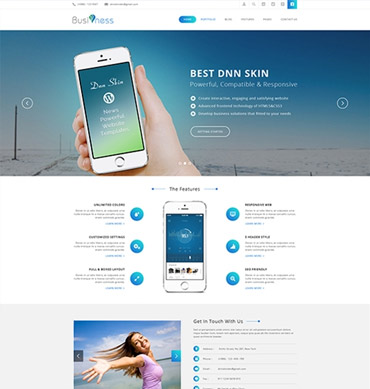A detailed description of a webpage being displayed on a computer screen is captured. The webpage prominently features the word "BUSINESS" where "BUSI" is colored in gray and "NESS" in blue. A teardrop-shaped icon is centered between the words. The interface includes various selections, with the first selection highlighted in blue, although the text is too small to decipher.

In the middle of the screen, a hand holds a smartphone displaying the message "best DNN skin," which is also the main headline on the webpage. Next to this image is a gray sidebar. The remaining visible webpage has a blue background featuring six paragraphs of text accompanied by blue dots with icons, though the writing is too small to read.

At the bottom of the webpage, a longer gray rectangular box contains a photograph of a young girl with long brown hair blowing in the wind. She is standing on a beach, wearing a purple top, extending her hand outward. The ocean and sky provide a serene backdrop. Surrounding the image are six blue bullet points containing text that is illegible due to its small size.